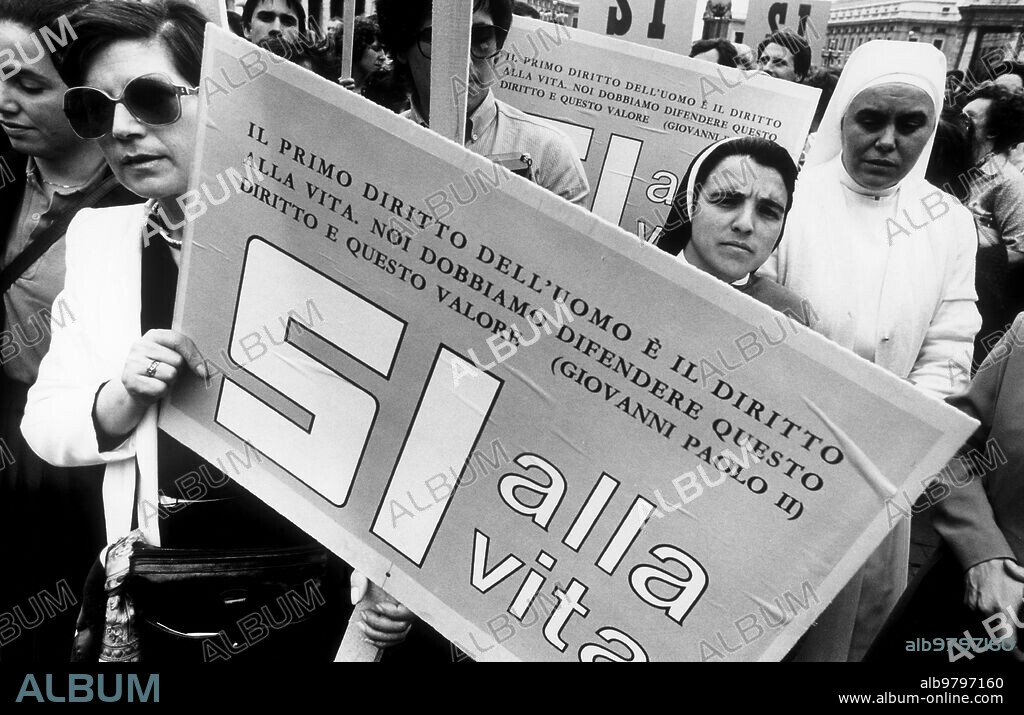This black-and-white photograph, marked as a stock image, features a prominent watermark reading "ALBUM" in alternating white and gray, alongside a lower-right text that includes "ALB9797160" and the website "www.album-online.com". At the very bottom, "album" appears in blue on a black background.

Central to the image is a man on the left, wearing sunglasses and a white blazer over dark clothes, holding a protest sign. The sign, written in Italian, states: "Il primo dorito dell'uomo è il dorito alla vita. Noi dobbiamo difendere questo dorito e questo valor. Giovanni Paolo II." The sign's large bottom text reads "SI ALLA VITA". The man grips the sign's edge with his right hand and its wooden handle with his left.

To the right of the man, walking directly towards the camera, are two women dressed as nuns. The nun on the left wears a traditional black habit, while the one on the right is clad entirely in white. Their expressions convey a sense of urgency and determination. The background reveals more people, potentially fellow protesters, blurring the distinction of individual roles but collectively emphasizing the march's purpose.